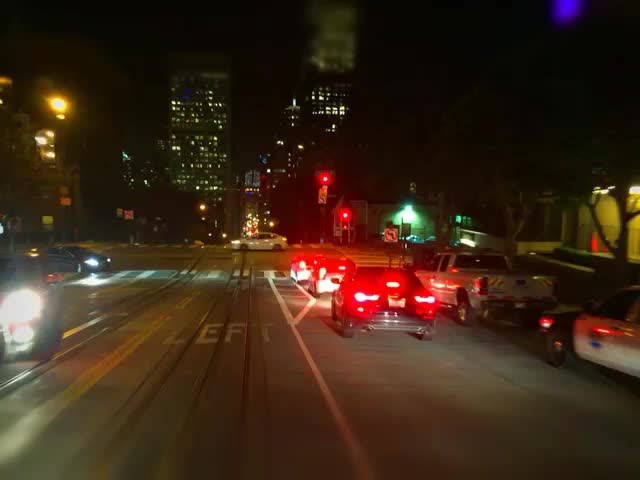The nighttime image captures a bustling street scene that appears to be on the outskirts of a major city, possibly New York. The black sky serves as a backdrop to several tall buildings, likely office structures, which are illuminated and at least 100 stories high. On the right side of the picture, five vehicles—three cars, a taxi, and a pickup truck—are halted at a red light. Their tail lights create a stark contrast against the darkness. 

To the left of these vehicles, there is a lane marked for left turns, delineated by a yellow line on the left and a white line on the right. Smaller buildings and various dark green trees can be seen along the street. Across the road, additional vehicles are approaching. There also appears to be a crosswalk nearby. Further in the background, the street seems to become busier, perhaps leading deeper into the city. A green traffic light is visible back there, and the area is cluttered with what might be trash and safety cones.

A single blue beam of light shines faintly from the top right corner of the image. The road may have tracks for cable cars, suggesting the possibility of San Francisco as the location. Overall, the cityscape is devoid of people but filled with vehicular activity, painting a vivid picture of urban life at night.